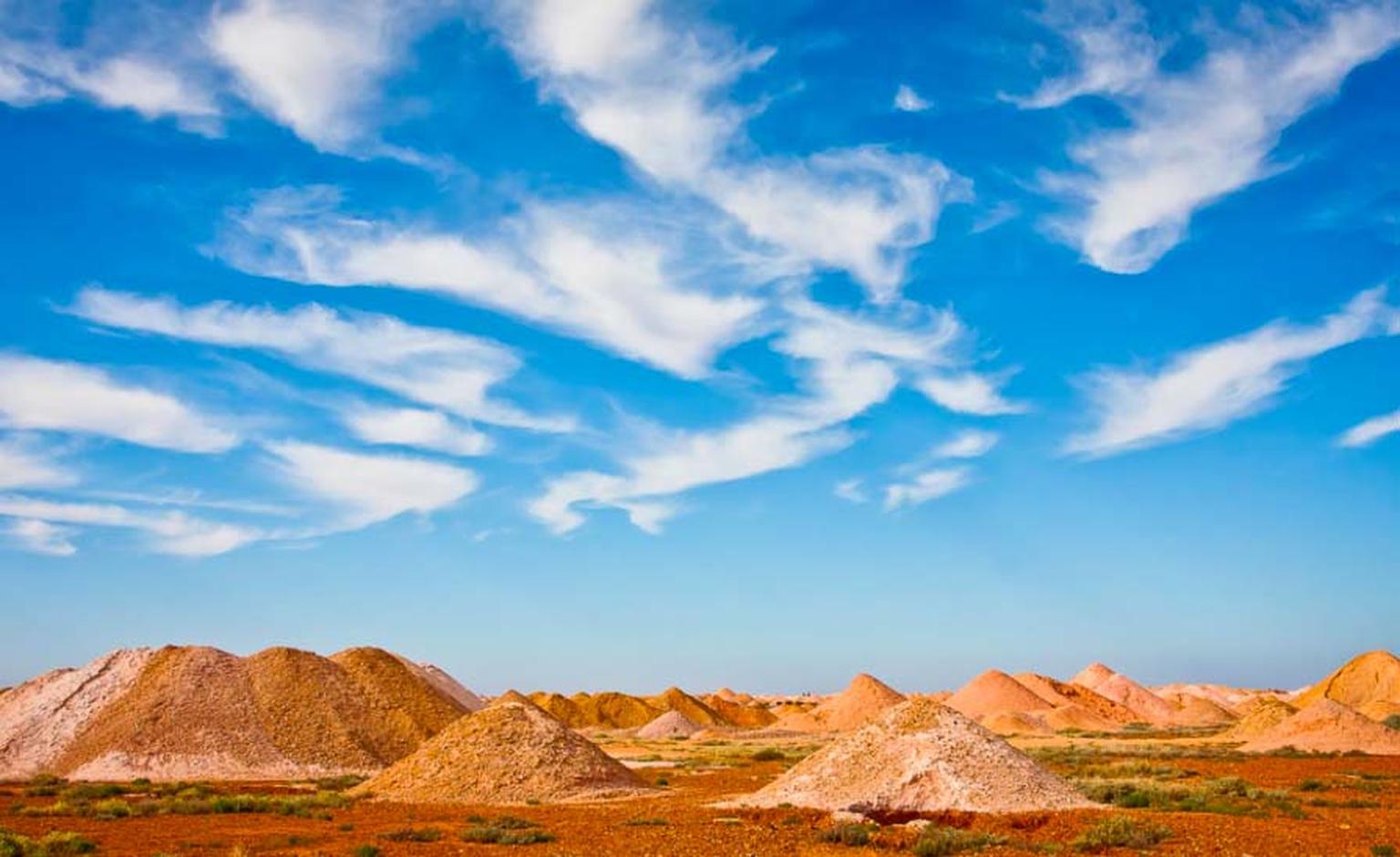The outdoor image showcases what appears to be a desolate desert scene with mounds and hills of sand and soil. The terrain is characterized by an intriguing mix of orangey-tan sand dunes and reddish soil mounds, some coming to distinct points. Scattered across this arid landscape are patches of sparse, scrubby greenery, adding a touch of life to the barren expanse. The sky, which occupies about two-thirds of the horizontal, rectangular photo, transitions from a light blue at the horizon to a more intense blue at the top, dotted with high, large, wispy clouds. The scene is free of any people or vehicles, leaving the viewer to focus solely on the natural elements captured in the image.